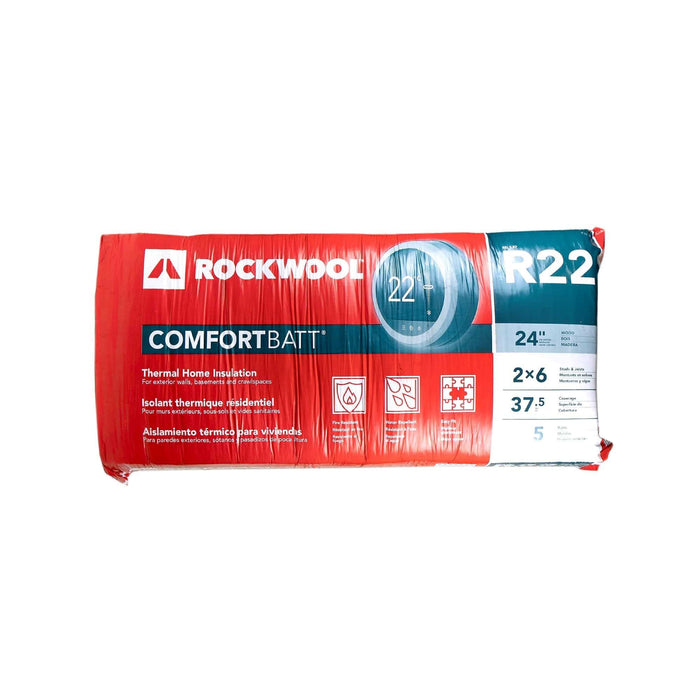The image displays a plastic-wrapped package of Rockwool insulation, predominantly red in color with a section in dark blue on the top right. The package features a white square on the top left with two facing red trapezoids. Adjacent to this square, "Rockwool" is prominently printed in white text. Below this, against a black bar, the words "Comfort Bat" are displayed, accompanied by a circular emblem with the number 22 inside it. Further down, the product is described as "Thermo Home Insulation," with translations in Spanish, "Aislamiento Térmico Residencial," and French, "Isolant Thermique Résidentiel."

On the right side of the package, there are three icons indicating fire resistance, water resistance (depicted by droplets), and interlocking puzzle pieces suggesting the ease of installation. Additionally, a dark blue box on the top right corner of the package states "R-22," with "24 inch" in lighter blue beneath it, followed by "2 by 6" and "37.5" indicating dimensional specifications.

In summary, this Rockwool insulation package includes markings that suggest its effectiveness for thermal home insulation, ease of application, and coverage area, making it suitable for residential use.